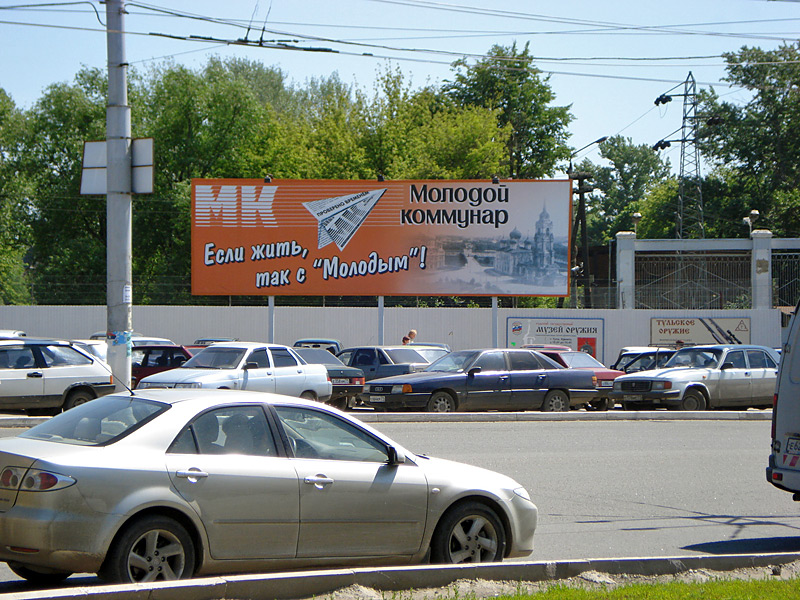The image depicts a bustling street scene, likely in Russia or an Asian country, featuring two lanes of traffic divided by a median. In the foreground on the right, a brown or beige sedan is parked by the curb. On the opposite side, numerous cars, including blue, silver, and white vehicles, are both parked and moving along the road. A significant backdrop includes a parking lot with approximately 20 cars. A prominent white wall stands behind this lot, adorned with a green billboard displaying a paper airplane made from a newspaper and the logo "MK," along with black and white Russian text. The top of the billboard features additional orange signage. The scene is framed with many tall, green trees and is further detailed with power lines and poles. The sky is clear and blue, lending an airy and open atmosphere to the street. The image also features a small grass patch at the bottom right, adding a touch of nature to the urban landscape.